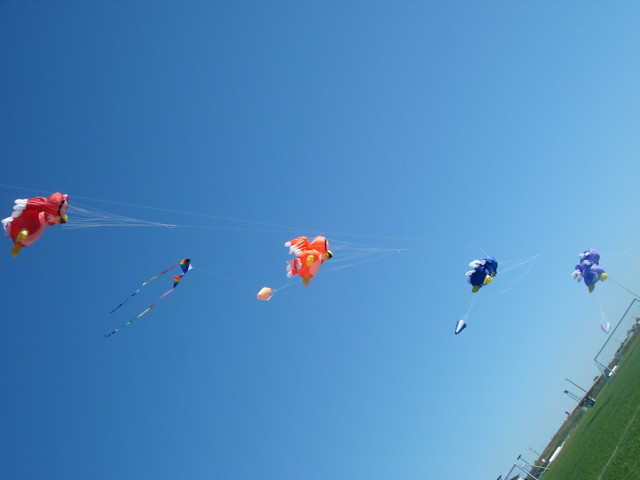The photograph captures a vibrant outdoor scene dominated by a clear blue sky, with no clouds in sight, and the sun casting light from an early morning angle. The image is taken at an angle, positioning the sky in the left-hand side and the green grass in the lower right-hand corner. Scattered across the sky, there are four kites flying in a horizontal line, each appearing to be linked by barely visible strings. The highest kite on the left is red, resembling a bird with a yellow and white edge. Moving right, the second kite is rainbow-colored with streamers trailing behind it. Below that, an orange kite with pale orange round appendages follows. Next is a dark blue kite, also featuring some roundish objects, and the kite closest to the ground is a lighter blue, almost translucent due to the lighting with similar white-tipped wings. On the ground, a lush green field is visible, with sports equipment such as a goalpost suggesting the setting of a soccer field. The kites add a whimsical contrast against the serene sky and green field, suggesting an atmosphere of leisure and joy.